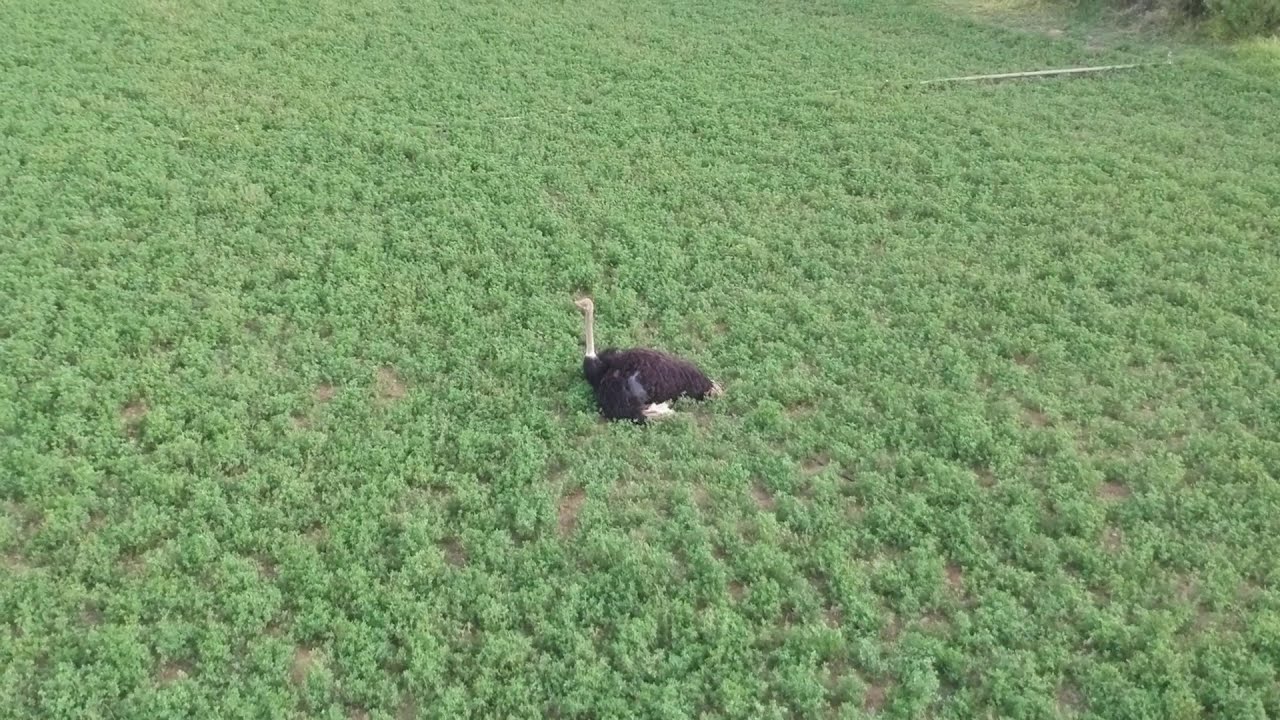This high-angle color photograph, taken in landscape orientation, features a lush field of vibrant green plants resembling small bushes, densely packed across the terrain. At the center of this verdant expanse is a large bird, which is seated upright but with its body grounded, suggesting it is an ostrich. 

The ostrich displays distinct coloration; its neck, head, and beak are tan, while its body is adorned with dark, blackish-brown feathers. Its legs are obscured from view as it rests on the grayish-brown earth visible between the plant clusters. The ostrich's posture includes its head and neck held high, pointing to the left of the image.

A subtle detail in the upper right corner of the photograph includes a small, nearly hidden pipe running horizontally, adding a touch of variety to the natural scene. The overall composition suggests a realistic, drone-captured depiction, with colors primarily in shades of green, brown, black, and tan. The image provides no other discernible objects or text, focusing solely on the tranquil, natural setting and the prominent ostrich at its heart.